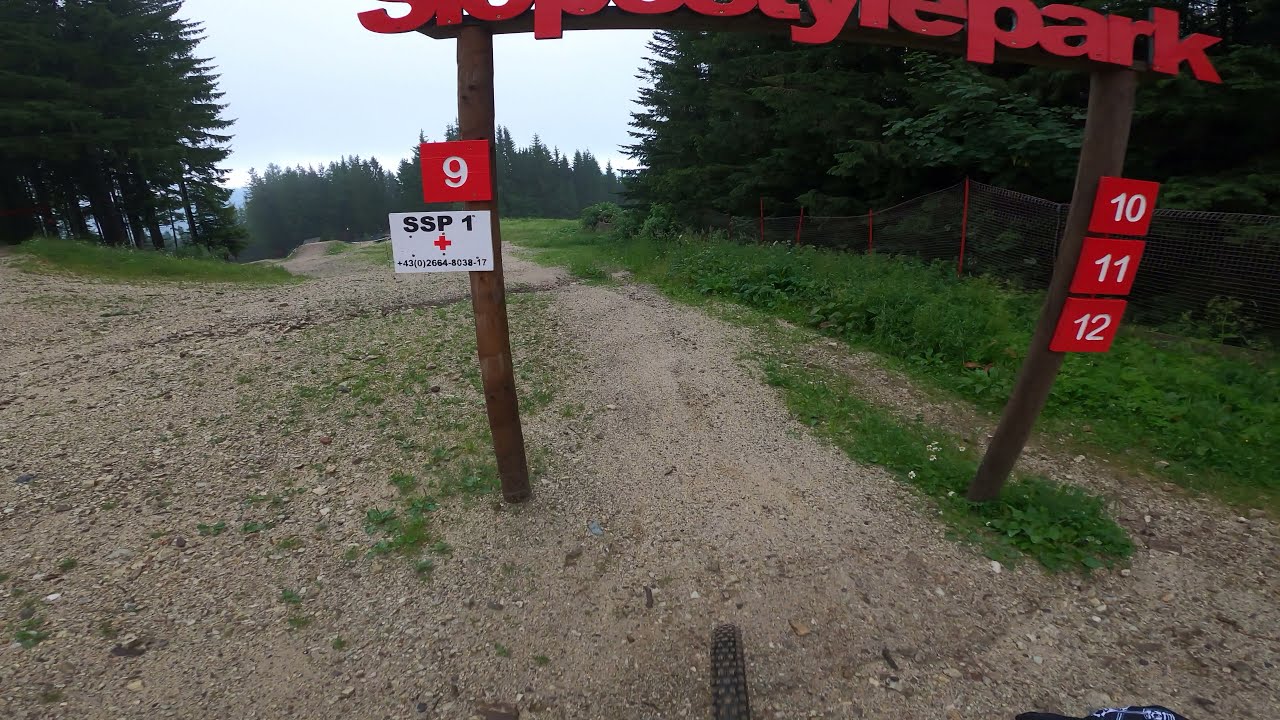The image captures a natural outdoor scene set in a public park, looking down a gravelly trail framed by trees, including several tall pine trees in the distance. Dominating the center is a wooden structure with vertical posts, suggesting a gateway or marker. While the complete text in red letters at the top of the structure is not fully visible, it ends with the word "Park". Below the sign, a mountain bike tire is placed at the bottom center of the frame, indicating preparation to traverse the path ahead.

To the left of the structure, a red square sign features the white number '9'. Beneath it is a white rectangle with black letters "SSP 1" and a red cross with some illegible black lettering below it. On the right side, three stacked squares display the numbers '10', '11', and '12' in white on a black background, possibly indicating checkpoint markers for a race or a trail route.

The ground beneath the structure is a mixture of sand and gravel, adorned with small stones and patches of low vegetation. A defined trail, slightly clearer of larger rocks, extends into the distance, flanked by periodic low-level plants. The scene is slightly darker, possibly suggesting an evening setting, and the trail leads off into the more densely wooded area, inviting exploration.